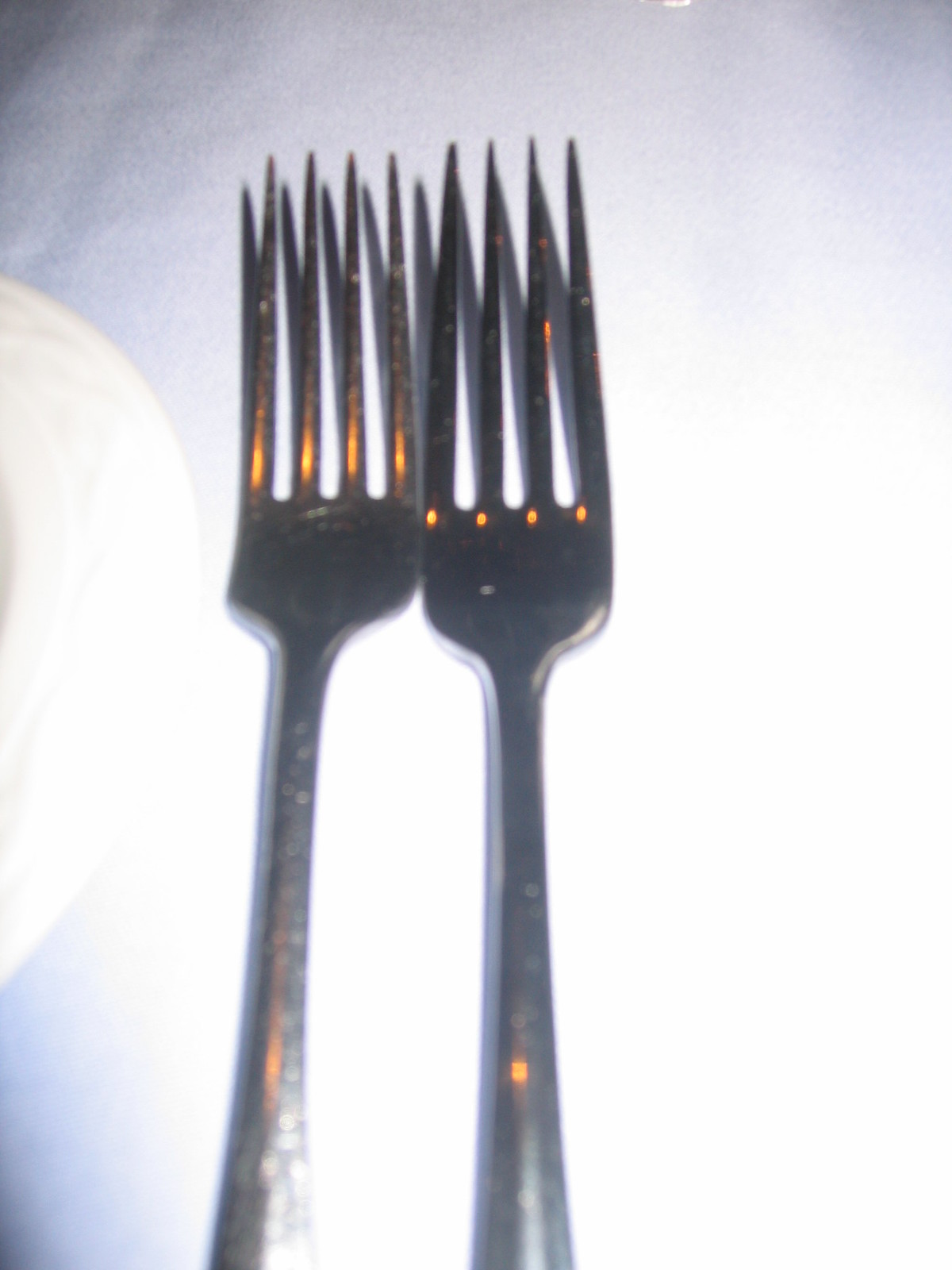This photograph captures a close-up, top-down image of two simple, stainless steel forks lying side by side on a white tablecloth, likely in a restaurant setting. The forks, which have four prongs each and lack any decorative engravings, appear almost identical and are positioned close to each other, with their tines and handles partially visible. The lighting is extremely bright, most likely due to a camera flash, casting a strong, reflective glare that creates a golden-orange tint on parts of the forks and intensifies the brightness of the white tablecloth beneath them. This lighting also produces distinct shadows beneath the tines, giving the impression of additional prongs. The photograph is blurry, particularly the fork on the left, and there is an indistinct, possibly spherical object (maybe a plate or saucer) on the left side of the frame, adding to the overall simplicity and minimalism of the scene.